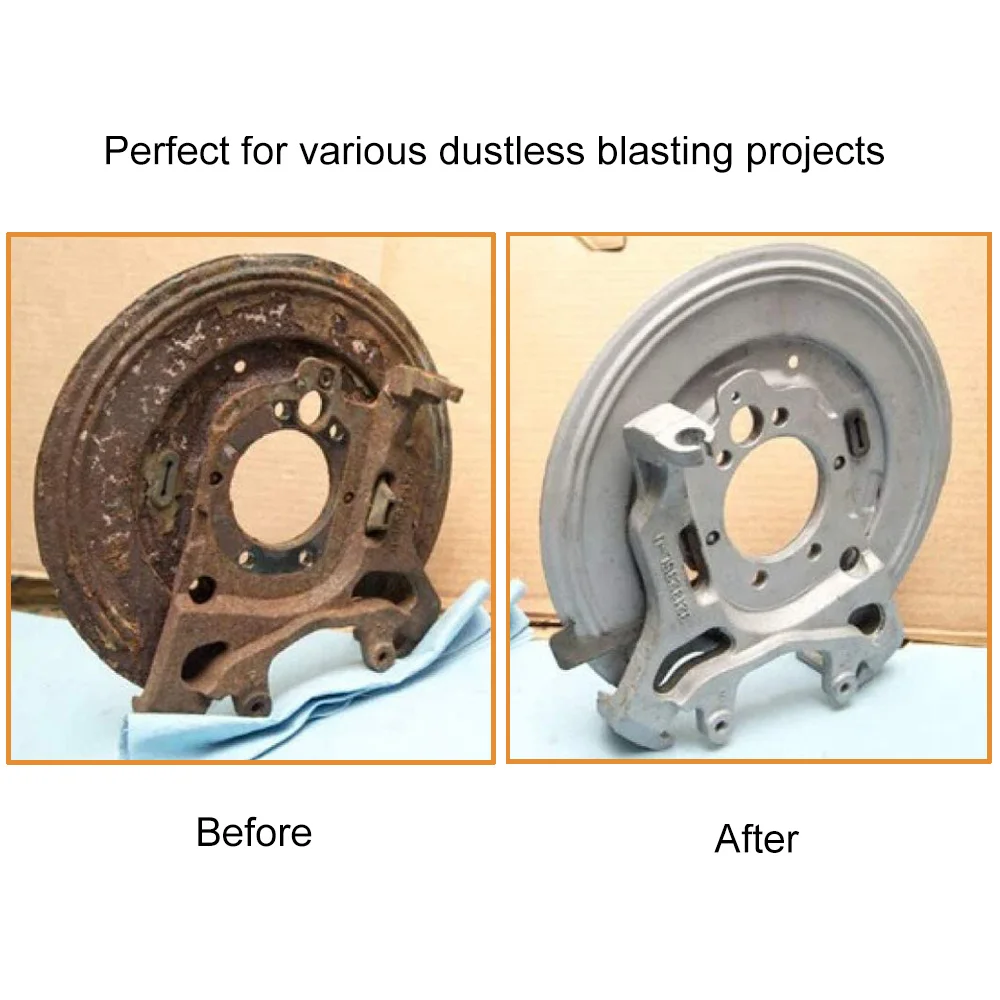This image showcases a dramatic before-and-after transformation, ideal for various dustless blasting projects. The top of the image features the caption in black text reading, "Perfect for various dustless blasting projects." Below, there are two side-by-side photographs: on the left is the "before" photo, displaying a heavily rusted and distressed mechanical part, likely steel, which appears as though it had been neglected and left out in the rain. This rusted item rests on a bunched-up blue cloth over a tan surface. The right side of the image presents the "after" photo, where the same part has undergone thorough cleaning and dustless blasting. It now gleams with a silvery, polished finish, nearly unrecognizable from its former state. This cleaned part sits on a smooth flat surface but still atop a blue cloth. Both images are framed with a cardboard background, emphasizing the stark contrast between the corroded and revitalized states of the mechanical part.